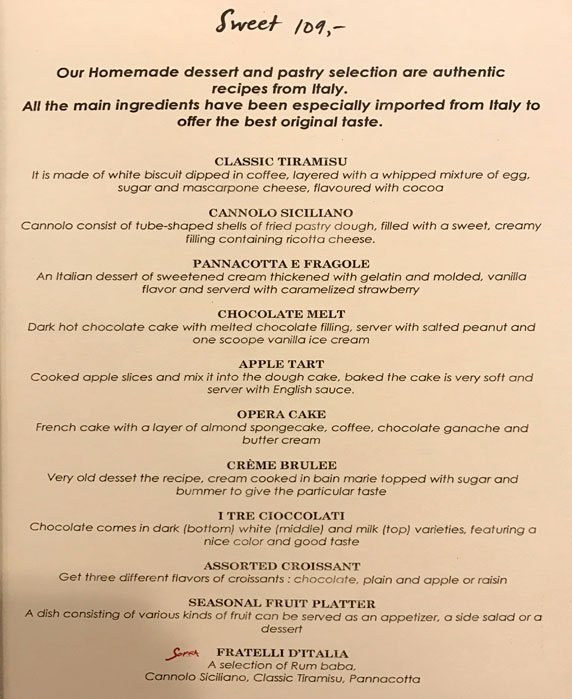The image depicts a dessert menu from an Italian restaurant. The menu, set against a piece of yellow paper with black text, features a handwritten-like font at the top that reads "Sweet 109." This could possibly indicate the price or a category title. Below it, there's a statement that reads: "Our homemade dessert and pastry selection are authentic recipes from Italy. All the main ingredients have been especially imported from Italy to offer the best original taste." The detailed list of desserts includes:

- **Classic Tiramisu:** Made with white biscuit dipped in coffee, layered with a whipped mixture of egg, sugar, and mascarpone cheese, and flavored with cocoa.
- **Canolo Siciliano:** Tube-shaped shells of fried pastry dough filled with a sweet creamy filling of ricotta cheese.
- **Panna Cotta e Fragiole**
- **Chocolate Melt**
- **Apple Tart**
- **Opera Cake**
- **Crème Brûlée**
- **Assorted Croissant**
- **Seasonal Fruit Platter**

At the bottom, the menu also features the phrase "Fratelli di Talla."